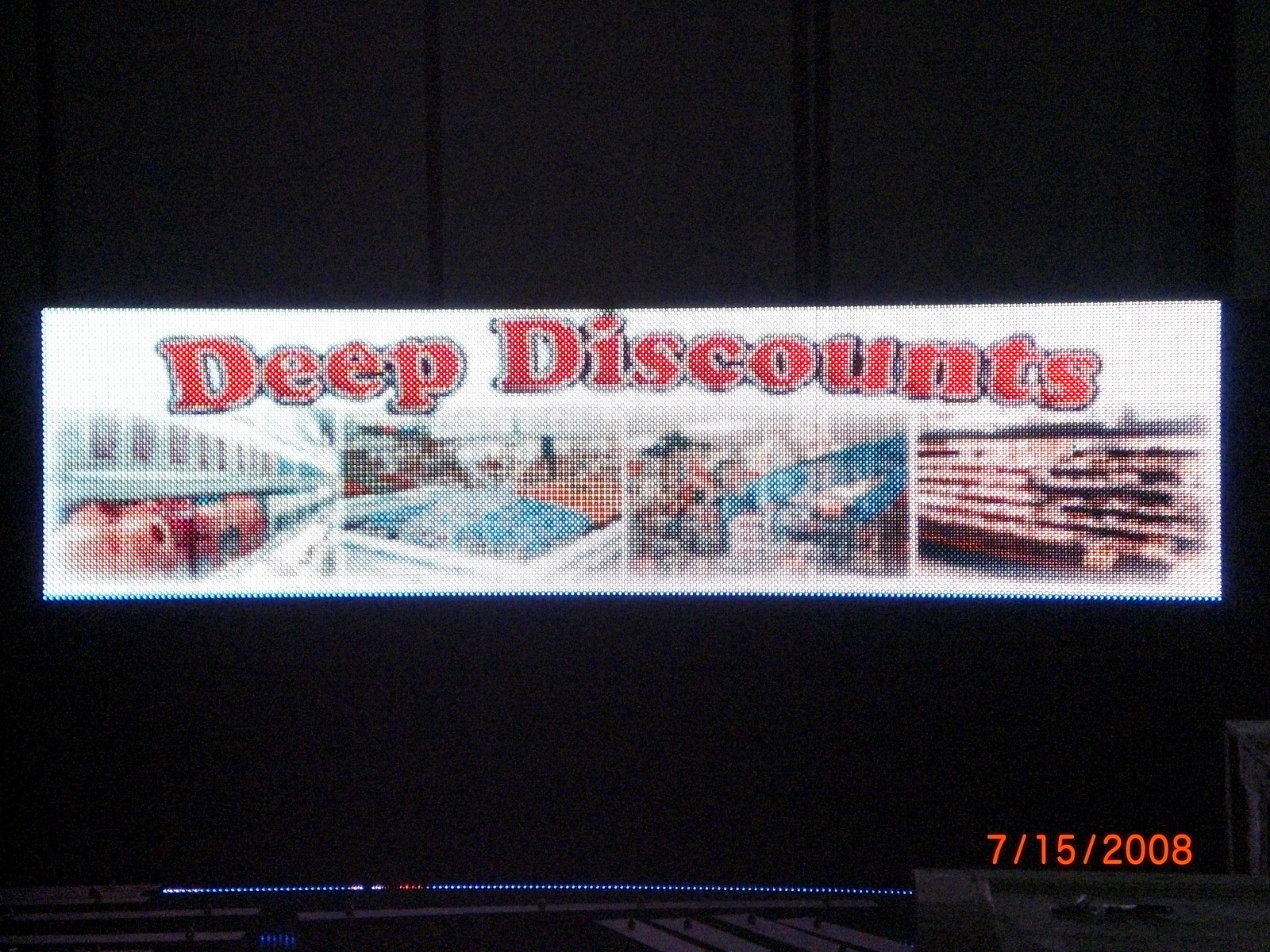The image is a low-resolution, black photograph taken at night, capturing a television displaying a pixelated advertisement. Dominating the center of the ad is a bright white background with the text "Deep Discounts" prominently displayed in red letters. The advertisement is segmented into four panels, each displaying indistinct images likely depicting various sections of a supermarket, including grocery shelves and large jugs of detergent, while one panel possibly shows produce bins. The majority of the image is shrouded in black, contributing to the overall blurred effect. At the bottom of the image, a sequence of blue, white, and orange LED-like dots stretches horizontally, adding a patterned detail. In the bottom right corner, the date "7-15-2008" is stamped in orange, marking the photograph’s timestamp.